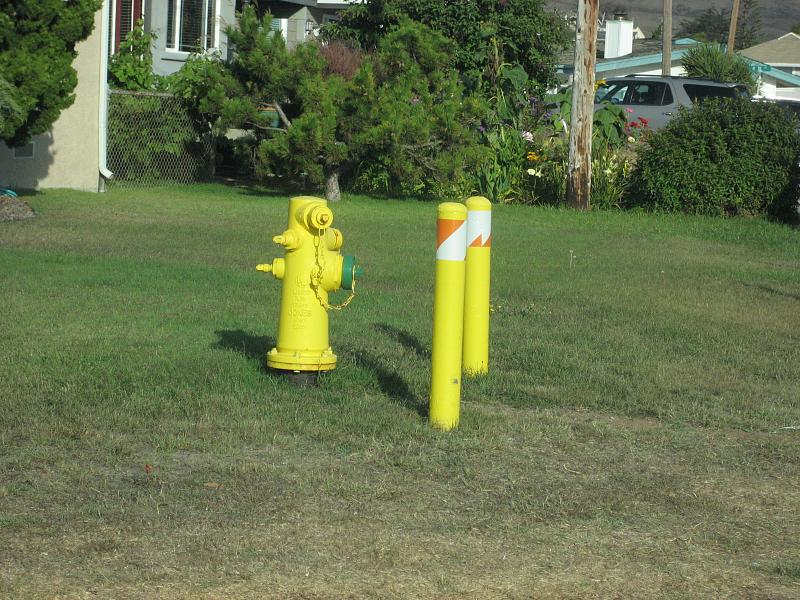In this detailed photograph, we see a green lawn peppered with patches of dead grass, indicating a hot summer day. Central to the image is a vibrant yellow fire hydrant, equipped with a green cap at the water outlet, connected by a yellow chain to the top of the hydrant. Flanking the hydrant to its right are two robust yellow poles, each with orange and white bands painted at their tops, seemingly designed to protect the hydrant. Behind this grouping, lush green trees and bushes partially obscure a silver fence and several townhouse-style single-family homes. A blue SUV is parked amid the greenery to the right. This image captures the tranquil yet functional aspects of a residential neighborhood.